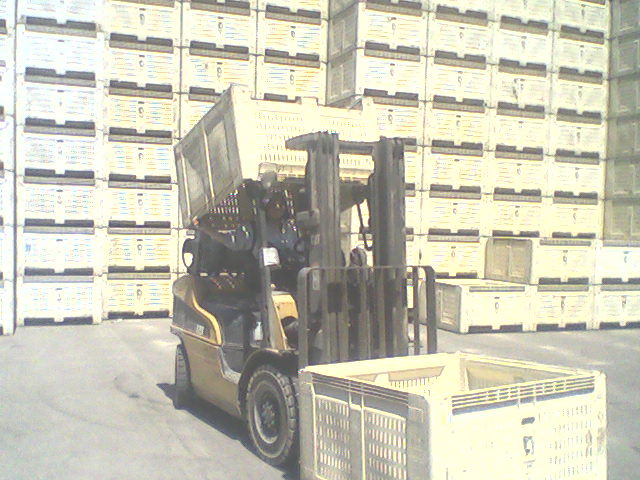The image depicts a small, yellow forklift in an outdoor cement area. The forklift is transporting a large, yellow plastic crate with an open-ended design reminiscent of a milk crate, complete with holes or vents on the sides. A similar crate is perched atop the forklift's cab, potentially placed there for shade. The forklift is operated by a Caucasian individual wearing a light blue shirt. The background is dominated by two large stacks of these crates, each towering at least 8 to 10 high and extending many rows across, suggesting the presence of several hundred crates. The image, seemingly overexposed with excessive brightness and contrast, appears to capture the scene either in a construction yard, shipping center, or distribution warehouse.